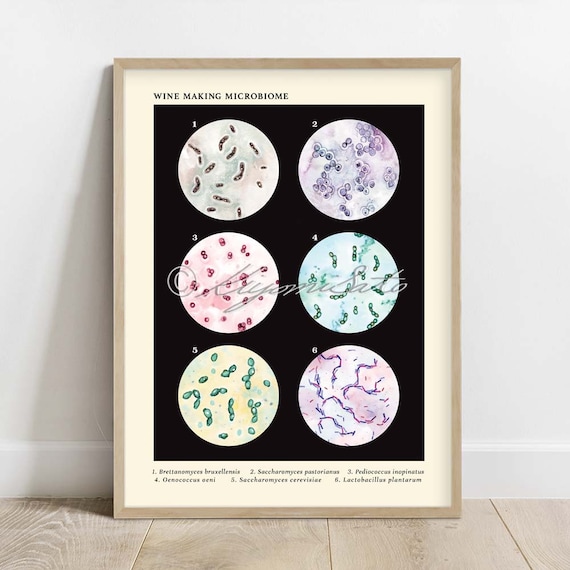The image depicts a detailed, framed picture leaning against a plain white wall on a tan or wooden floor. The picture is centered around the concept of the "Wine Making Microbiome," prominently displayed in elegant cursive at the top. Below this, the black background features six distinct circular diagrams, each representing different microbes involved in the wine fermentation process. The microbes are illustrated in various shapes and colors—including shades of green, blue, yellow, red, gray, and purple—and are labeled with white numbers from 1 to 6. Each microbe illustration shows unique formations, such as bean shapes, clusters of circles, paired circles, rows of four circles, pea-shaped structures, and interconnected lines in purple and red hues. Beneath each circle, there is small black text with Latin names of the bacteria, detailing each stage of the microbiome. The entire visual is enclosed within a beige wooden frame, enhancing its informational yet artistic appeal.